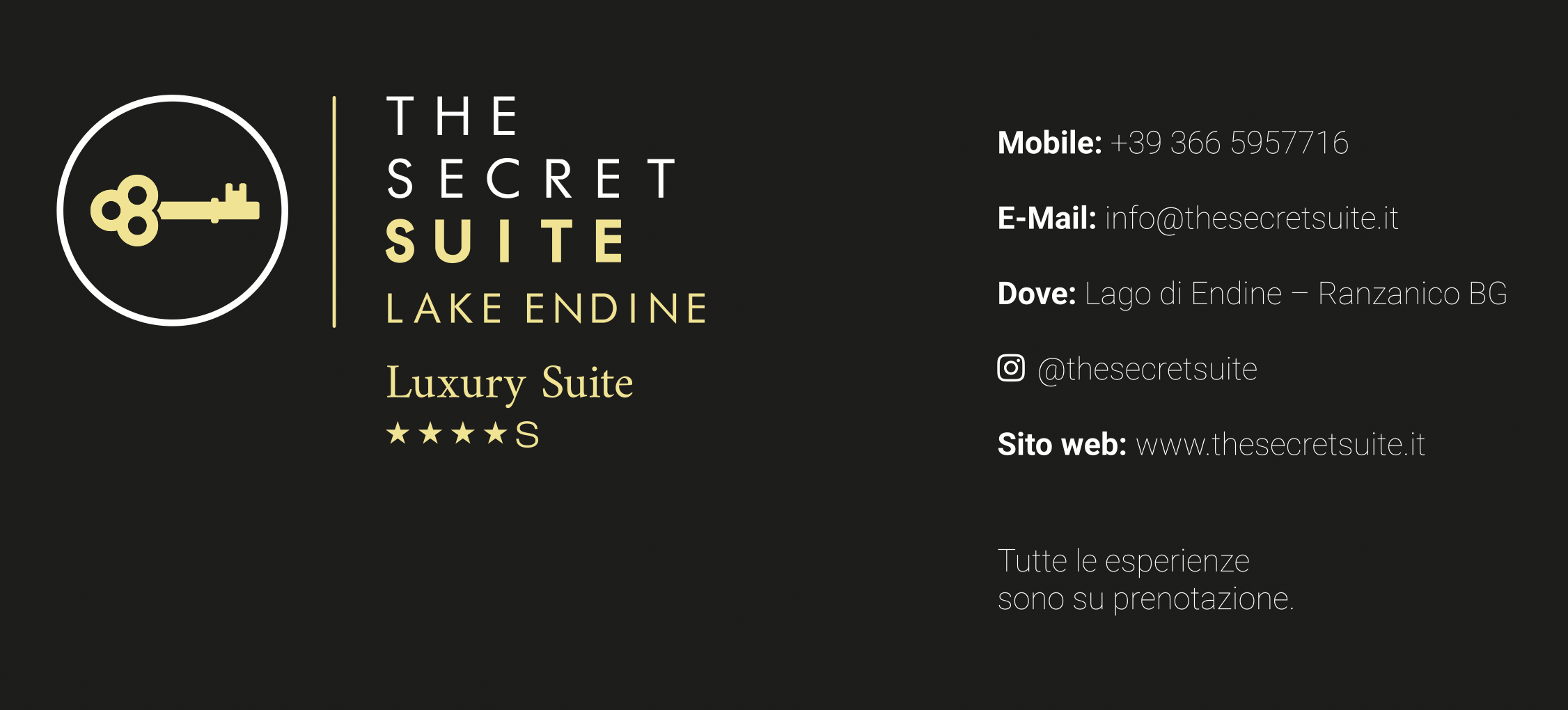This image depicts a business card with a sleek, elegant design. The background is entirely black, providing a sophisticated canvas for the information presented in white and gold colors. On the top left, a white circle encloses a gold key, symbolizing luxury and exclusivity. To the right of the key icon, the text reads "The Secret Suite, Lake Endine, Luxury Suite." Beneath this, four gold stars are followed by the letter 'S'.

On the right side, smaller white font details the contact information: "Mobile: +39 366 595 7716" and "Email: info@thesecretsuite.it". Further down, the location is specified: "Lago di Endine - Ranzanico, BG." Below this, there is an Instagram icon with the handle "@thesecretsuite," and the website "www.thesecretsuite.it". The card also includes an Italian phrase: "Tutte le esperienze sono su prenotazione," meaning "All experiences are by reservation."